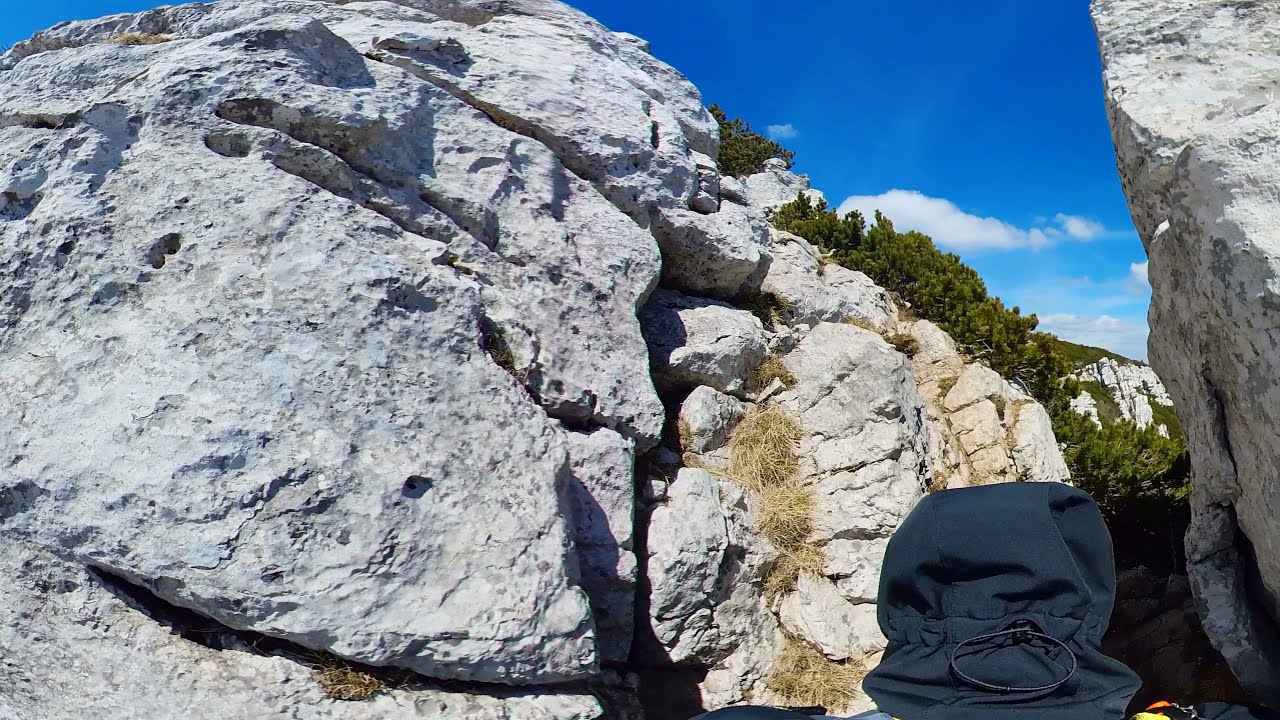This photograph captures a stunning view of a rocky formation, possibly a canyon or mountain valley. The tall, gray rock walls dominate the left and right of the image, where you can see small patches of yellowish hay or grass emerging from the crevices. Nestled between these towering cliffs is a vibrant display of green plant life, which includes evergreen trees and possibly bushes. The background features more of these rocky structures, forming a natural walkway that people could traverse. Above the breathtaking scenery, a bright blue sky stretches across the middle of the photo, adorned with fluffy white clouds. In the bottom right corner, someone wearing a navy-blue bucket hat or hoodie adds a subtle human element to the natural landscape. The light gray tones of the rock walls contrast beautifully with the lush greenery and clear sunny sky, making it a picturesque and serene scene.